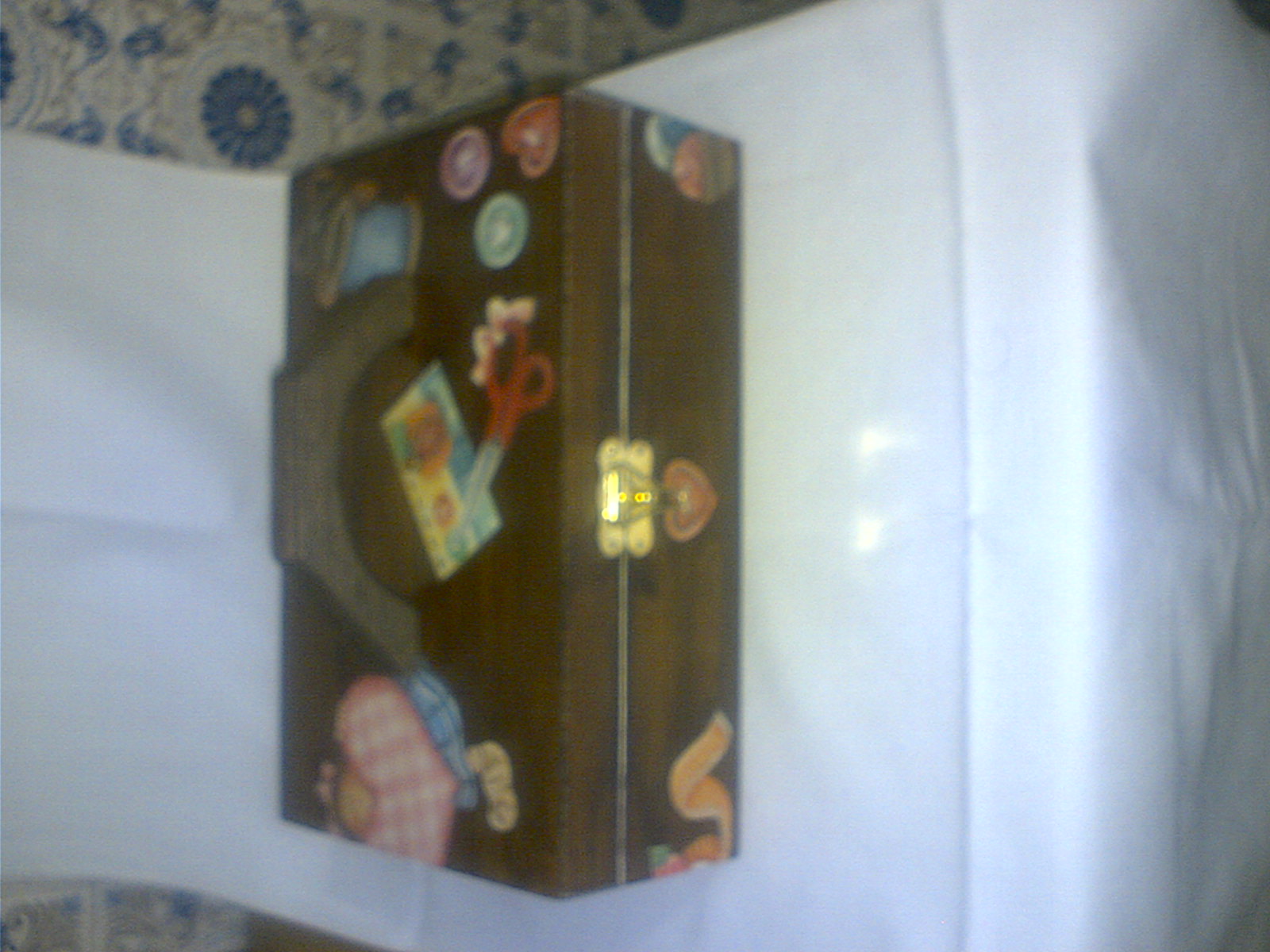The image features a slightly grainy, sideways photograph of a brown wooden box adorned with various colored graphics, stickers, and stamps, including images of scissors, hearts, and possibly a spool of yarn. The box, equipped with a gold latch and a wooden handle on top, is positioned vertically and slightly offset to the left, resting on a piece of white fabric that obscures the underlying surface. The background reveals bits of tan and blue floral-patterned wallpaper peeking out from the top left and bottom left corners of the image, suggesting the box is in a personal setting, possibly on a fabric-covered white chair. The overall perspective appears flipped counterclockwise by 90 degrees, making the objects run horizontally from left to right instead of the usual vertical orientation.